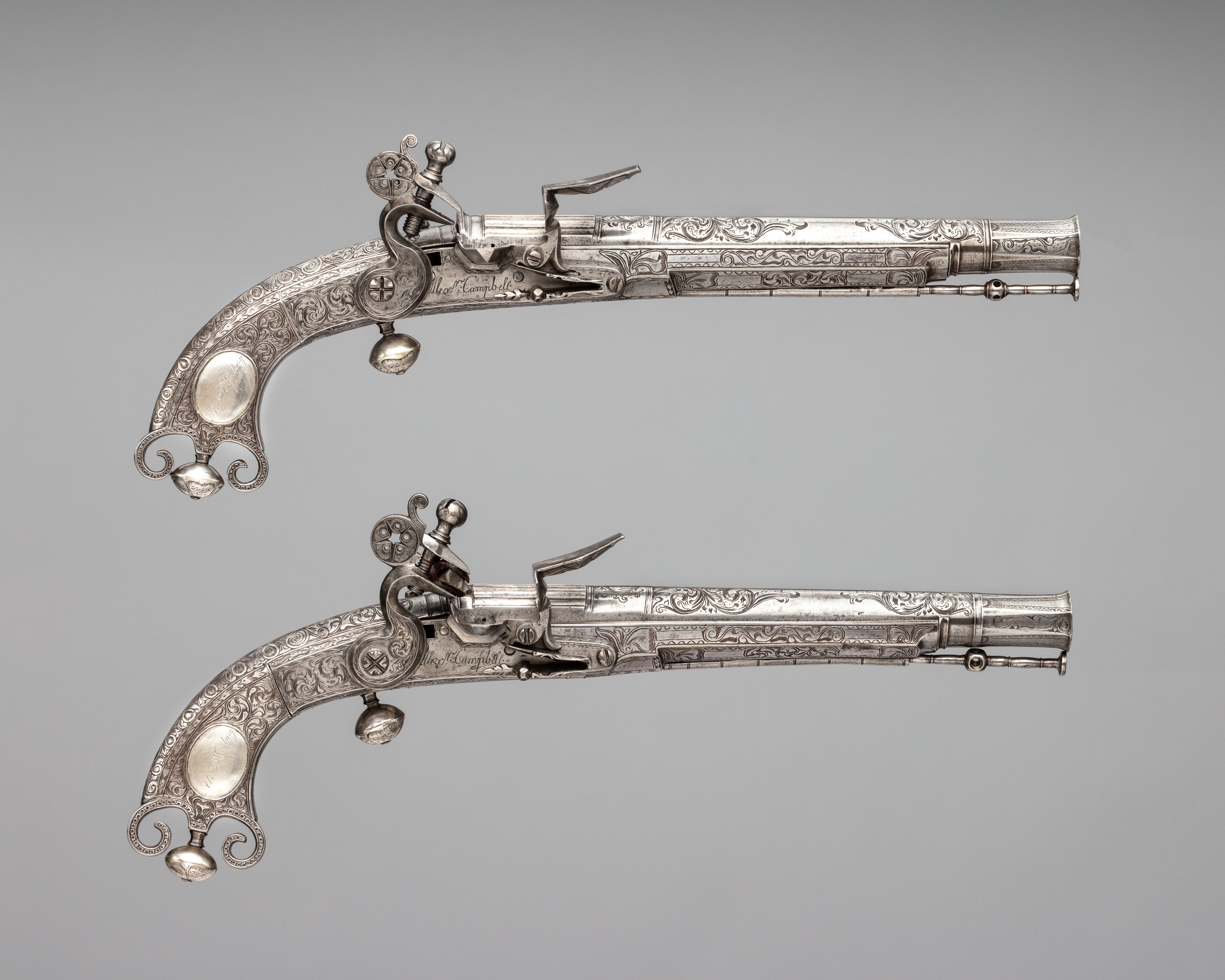This image showcases two near-identical, old-style revolvers, likely dating back to between the late 1700s and early 1900s. The guns are positioned one below the other on a light-to-dark gradient gray background, which smoothly blends from lighter in the center to darker towards the edges. These revolvers exhibit a highly ornate and intricate design, with elaborate etchings and carvings across their silver-colored metal bodies. Each gun features a pearl-like detail on the finely decorated handle and a latch mechanism on top, likely used for firing. The design is deeply detailed, making the revolvers appear both decorative and functional. The background remains plain with no additional text or items, ensuring full focus on the ornate and historical firearms.